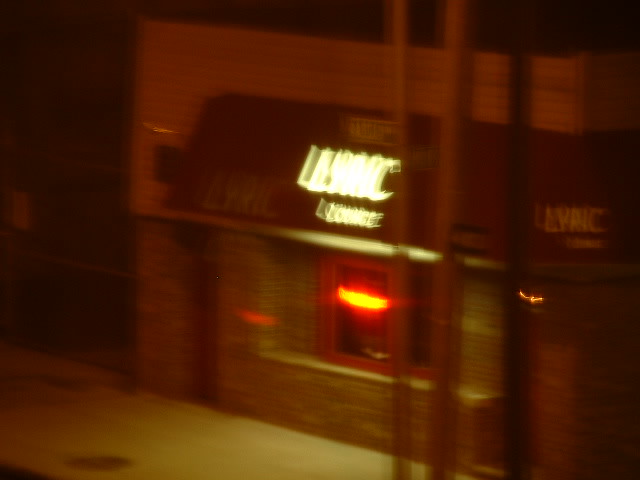This nighttime photograph captures the blurry facade of a brick building, identified as the Lyric Lounge. The motion blur suggests it may have been taken from an elevated, moving vehicle. Illuminated primarily by a nearby streetlight, the building features a prominently lit red fluorescent sign, though the text on it is indecipherable due to brightness. An overhang spans the entrance, displaying the name "Lyric Lounge" multiple times in lit-up signage. A visible sidewalk to the bottom left of the image shows a small pothole, and a gray fence or gate is connected to the building's left side. Further details include a street sign standing between the photographer and the building, several windows, a door, and what appears to be a ladder along the side. Despite the blur, this photo effectively captures the essence of the Lyric Lounge illuminated against the night sky.